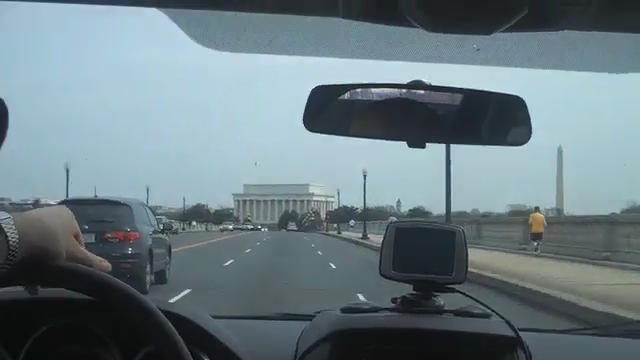The image captures a detailed scene within a vehicle, driving through Washington, D.C. In the foreground, the driver's silver watch with a metal clasp is visible as one hand rests atop the steering wheel. The rearview mirror and a dash-mounted GPS device are also seen. The interior of the car is dark-colored. Ahead, the road is a three-lane segment of a six-lane bridge, demarcated by white dotted lines, with sparse traffic. To the left, an Acura SUV either just passed or is about to be overtaken. The scene ahead is dominated by iconic landmarks: the Lincoln Memorial stands directly in front of the car, while the Washington Monument is slightly to the right. A sidewalk runs alongside the bridge, where a man in a yellow t-shirt and black shorts jogs. Periodic street lamps line the path, illuminating the overcast blue sky above.